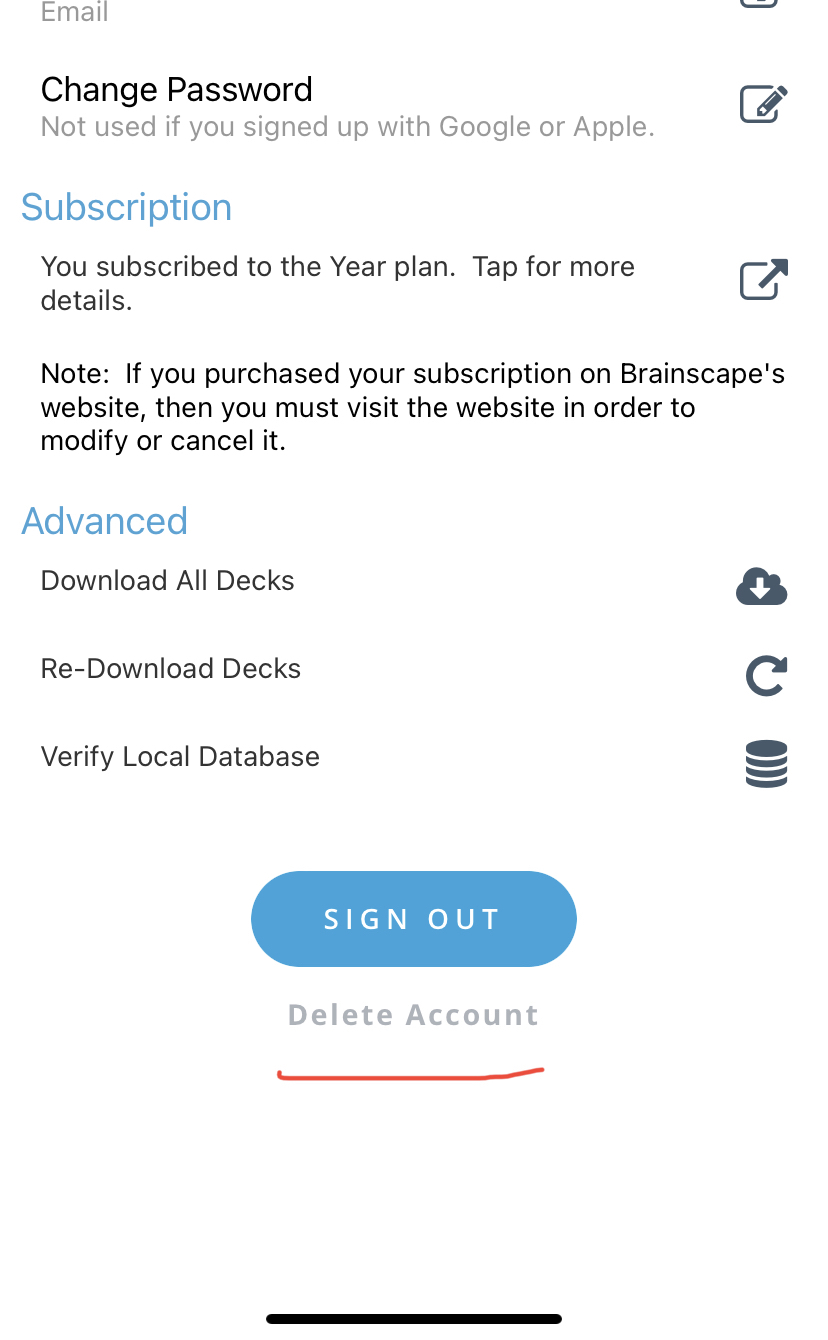This image presents a user interface screen with a white background and various sections related to email and account settings. 

- In the top-left corner, "Email" is prominently displayed, followed by the option "Change Password."
- Below that, there is a box featuring a pencil icon, suggesting an editable field.
- Further down, the word "Subscription" is highlighted in blue text. Additional information indicates that the user is subscribed to a yearly plan with a prompt to click for more details. Adjacent to this subscription detail is an icon box with an upward-right pointing arrow.
- A note clarifies that if the subscription was purchased via Brainscape's website, any modifications or cancellations must also be managed on the website.
- The next section, marked "Advanced" in blue text, includes options such as "Download All Decks" accompanied by a cloud icon with a downward arrow, "Redownload Decks" next to a circular arrow, and "Verify Local Database" with an icon of four stacked disks.
- Centered on the page is a prominent blue button labeled "SIGN OUT" in all capital letters, with white text.
- Below this button, again centered, is the "Delete Account" text underlined in red.
- The bottom of the page is defined by a black bar running across its width.